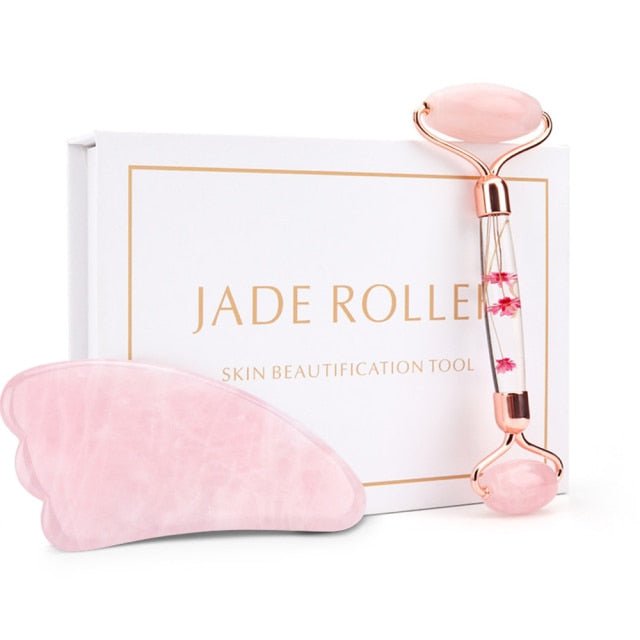This image features a white box with a gold frame in the center, containing the words "Jade Roller" in gold font, and beneath that, smaller lettering that reads "Skin Beautification Tool." Leaning against the box are two items: a jade roller and a gua sha tool. 

The jade roller consists of a clear handle filled with delicate pink flowers, and at each end of the handle, there are oval-shaped pink jade stones. One end of the jade roller has a larger stone, while the other end has a smaller one; these are used to massage the face and supposedly reduce puffiness and swelling.

Next to the jade roller is a gua sha tool, which is an oblong, foot-shaped piece of pink jade with notched edges designed for facial massage. This tool complements the jade roller for a full skin beautification routine.